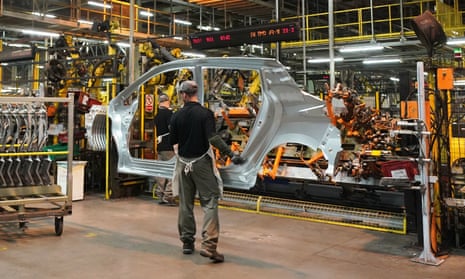This indoor photograph captures a bustling car manufacturing plant, characterized by its industrial environment and active machinery. At the center, a Caucasian man is seen from the back, his head slightly turned to the left. He is wearing a gray hat, a black short-sleeved polo with a green undershirt, long gray or khaki pants, a white apron, and brown boots. His right forearm is protected by a long glove. The man appears to be interacting with a large metallic car component, possibly a freshly stamped subframe or side panel of a sedan, displayed in an unfinished silver state. 

The setting features a complex arrangement of machinery and robotic arms involved in car part manufacturing. Above the scene, a catwalk with yellow railings and digital displays, featuring red and orange writing, add to the industrial ambiance. The flooring beneath the worker is light brown concrete, enhancing the utilitarian feel of the factory. Layers of metal platforms and various car part machines form the backdrop, emphasizing the continuous activity and the advanced manufacturing processes within this large warehouse. Although the background is somewhat blurred, the overall impression is one of a highly organized and operational car production facility.